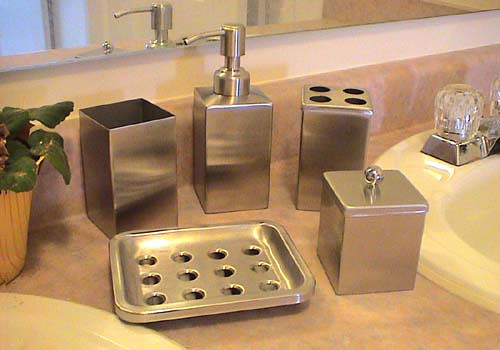The image depicts a meticulously arranged bathroom counter adorned with five silver containers. From left to right, the first container is a tall, lidless, rectangular vessel that appears empty. The central container at the back is a soap dispenser, distinguished by its silver pump top. Adjacent to it, on the right, is a rectangular toothbrush holder featuring four round openings on its lid. Positioned in the front right is a smaller cube-shaped container, topped with a silver lid adorned with a round ball handle, ideal for storing Q-tips or cotton balls. Below that is a soap dish designed with 12 holes for drainage, preventing soap from becoming mushy. The bathroom counter itself is topped with a beige marble-patterned surface.

A large mirror spans the entire length of the countertop, affixed to the wall above it. To the far left, a small houseplant with vibrant green leaves resides in a brown planter, adding a touch of nature to the scene. Two white sink bowls are partially visible, one in the lower left and more prominently the one on the far right. The sink fixtures are crafted from silver chrome and feature clear acrylic knobs, providing a modern touch to the overall design. The image does not contain any text.